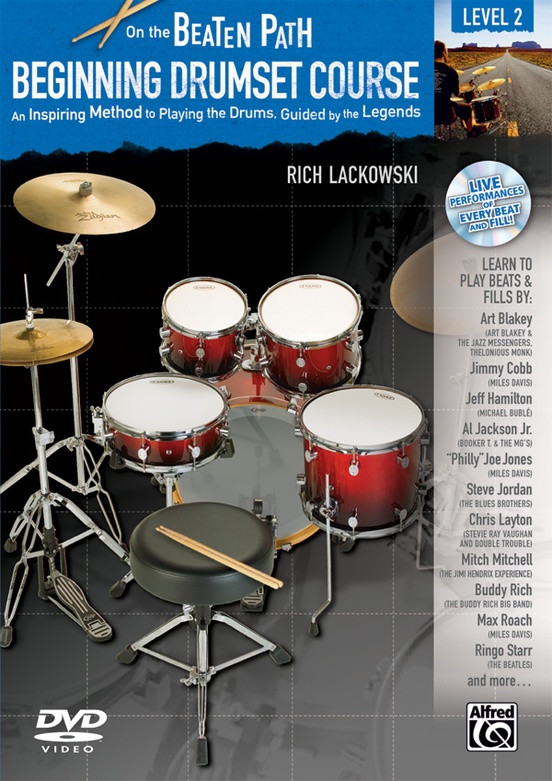The cover of this DVD, titled "On the Beaten Path: Beginning Drum Set Course," features a detailed image of a drum set. The drum set is predominantly red with darker maroon tones towards the bottom and is accompanied by brass cymbals on the left side. A black stool with four legs is placed at the front, with a pair of drumsticks laid across it. The cover's upper portion has a blue background with the main title in large white text: "On the Beaten Path." Below that, in all capital letters, is "BEGINNING DRUM SET COURSE," and further down in smaller writing is the subtitle, "An Inspiring Method to Playing the Drums, Guided by the Legends."

In the top right-hand corner, there is a blue banner with white text that reads "LEVEL 2." Below this banner, there is a depiction of a person playing drums on the road in a desert-like setting. The right side of the cover features a side banner listing names of legendary drummers such as Art Blakey, Jimmy Cobb, Jeff Hamilton, Philly Joe Jones, Mitch Mitchell, Buddy Rich, Max Roach, Ringo Starr, and more, with the caption "Live Performances of Every Beat and Fill."

Additionally, the bottom right corner features the Alfred logo in a black and white square. On the lower left, there's the DVD Video logo, indicating that this music book includes a DVD. 

The cover design is portrait and rectangular, giving a comprehensive visual experience of what the DVD offers to aspiring drummers.